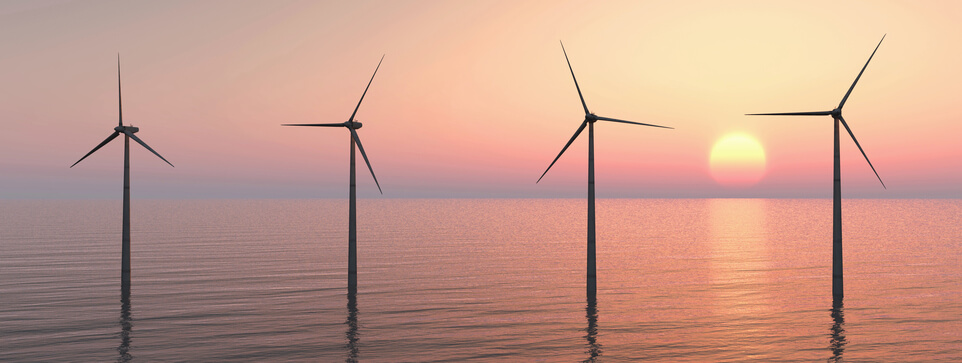The image captures four large offshore wind turbines lined up side by side in the tranquil ocean, each with three blades, made of gray metal. Their exact positions and whether they are currently spinning are indiscernible from the still photo. The serene water beneath them is remarkably calm with no waves, mirroring the peaceful ambiance of the setting. The backdrop features a breathtaking sunset, painting the sky and horizon with a blend of rich oranges, reds, pinks, and yellows. A gradient of colors, ranging from medium blue at the horizon to the pink hues reflecting off the ocean's surface, enhances the stunning vista. The harmonious contrast between the serene ocean, the industrial windmills, and the vibrant sunset creates a captivating and tranquil scene.